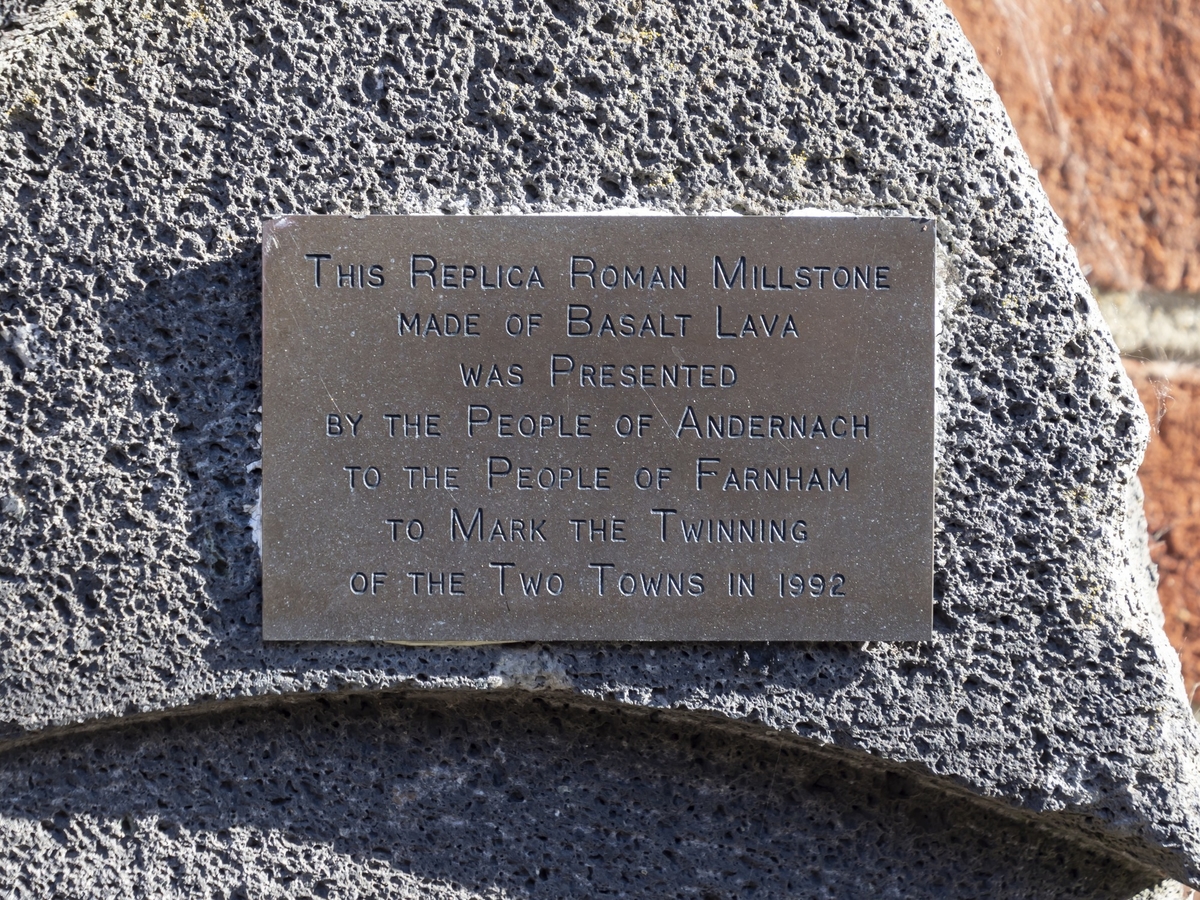This photograph captures a close-up of a gray, porous piece of basalt lava with a bronze plaque affixed to it. The inscription on the plaque reads, "This replica Roman millstone made of basalt lava was presented by the people of Andernach to the people of Farnham to mark the twinning of the two towns in 1992." The setting features a red brick wall in the background, suggesting the photo was taken outdoors on a sunny day. The bright sunlight creates a notable shadow that extends from the rim of the basalt lava towards the bottom of the image, emphasizing the stone's rugged texture and granular appearance.